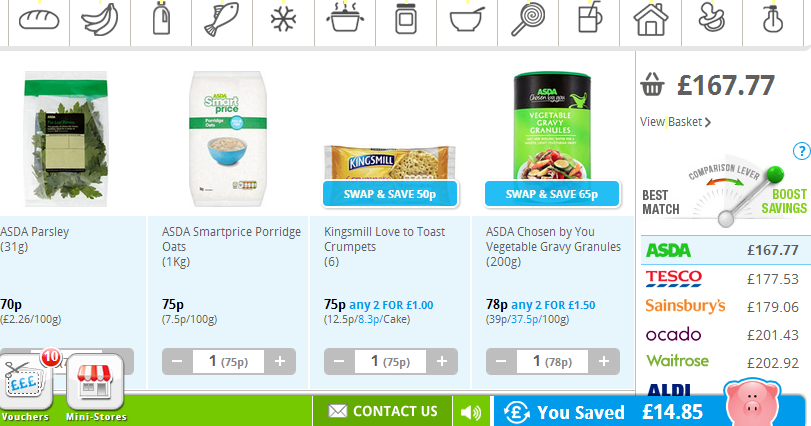The image appears to be a screenshot from a grocery shopping application or website. At the top of the screen is a taskbar featuring a series of icons representing various categories, such as a loaf of bread, a bunch of bananas, a milk jug, a fish, a snowflake, a steaming pot, a jar with a label, a bowl with a spoon, a lollipop, a glass with a straw, a house, a pacifier, and a light bulb.

Below the taskbar are four product images displayed in a row from left to right. The first image shows a bag labeled "ASDA Parsley" priced at 70p. The second image depicts a bag of "ASDA SmartPrice Porridge Oats." The third image is a package labeled "Kingsmill Love To Toast Crumpets." The fourth and final image displays a container labeled "ASDA Chosen By You Vegetable Gravy Granules."

On the far right of the screen, there is a section showing a shopping basket with a total amount of $167.77. Below this total, a lever-like element is labeled "Boost Savings." This section also lists various competing grocery stores—ASDA, Tesco, Sainsbury's, Ocado, Waitrose, and Aldi—along with the comparative prices of the items in the basket from each store.